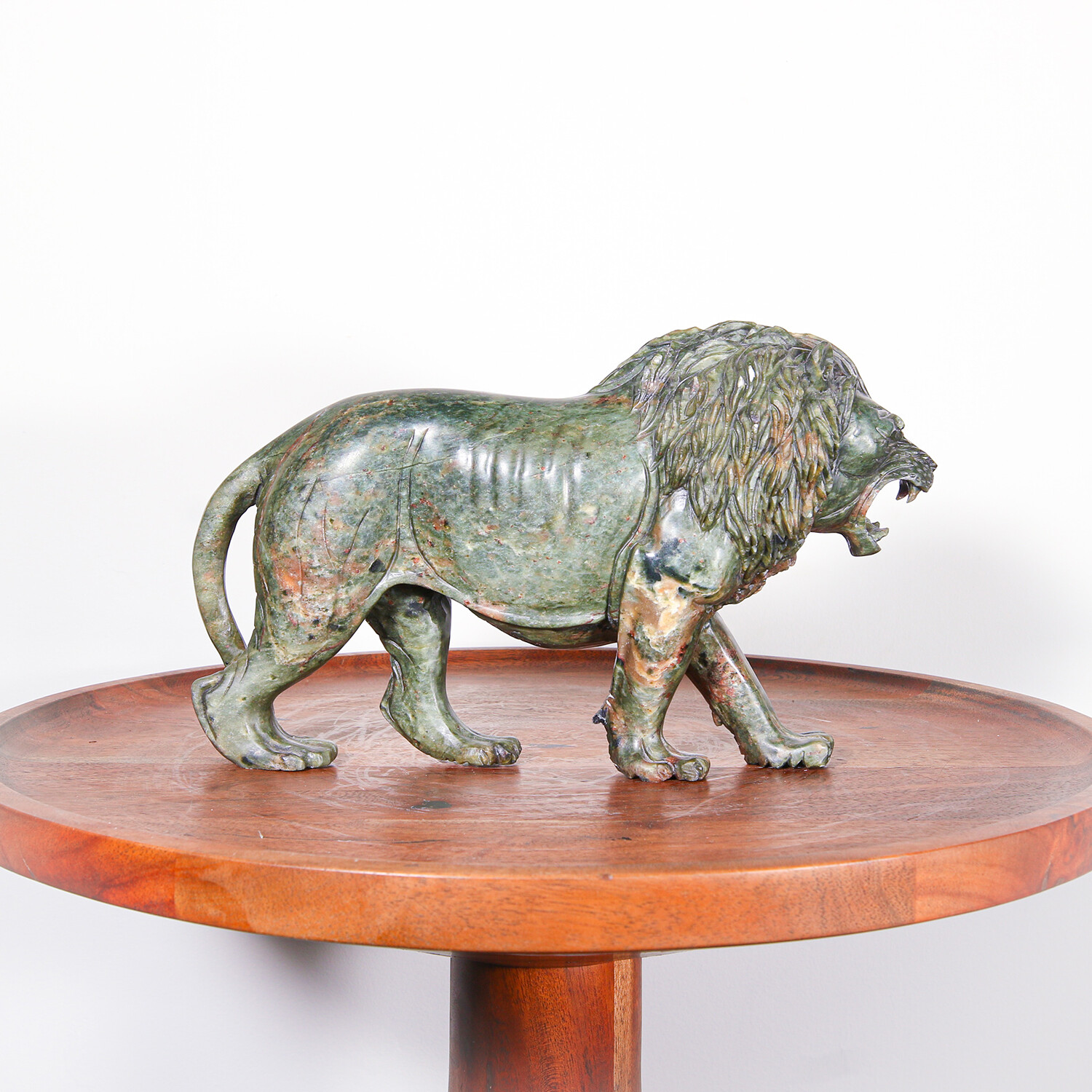The image depicts a highly detailed sculpture of a roaring lion, meticulously crafted from clay or a similar material with a patina giving it shades of olive green, copper orange, and hints of brown, black, and white. The lion is portrayed in a dynamic stance, facing to the right, with all four legs visible as if in mid-stride. Its large, intricate mane and sharp upper teeth paired with less prominent bottom teeth are strikingly visible. The sculpture, appearing almost miniature, rests on a small, round wooden table that is mahogany-colored. The table's pedestal base, also made of wood and matching the tabletop, supports the lion prominently. The photograph is taken against a pure white background, zoomed in to capture the detailed textures and vibrant colors of the lion and just the top of the table, emphasizing the statue’s artistic qualities.